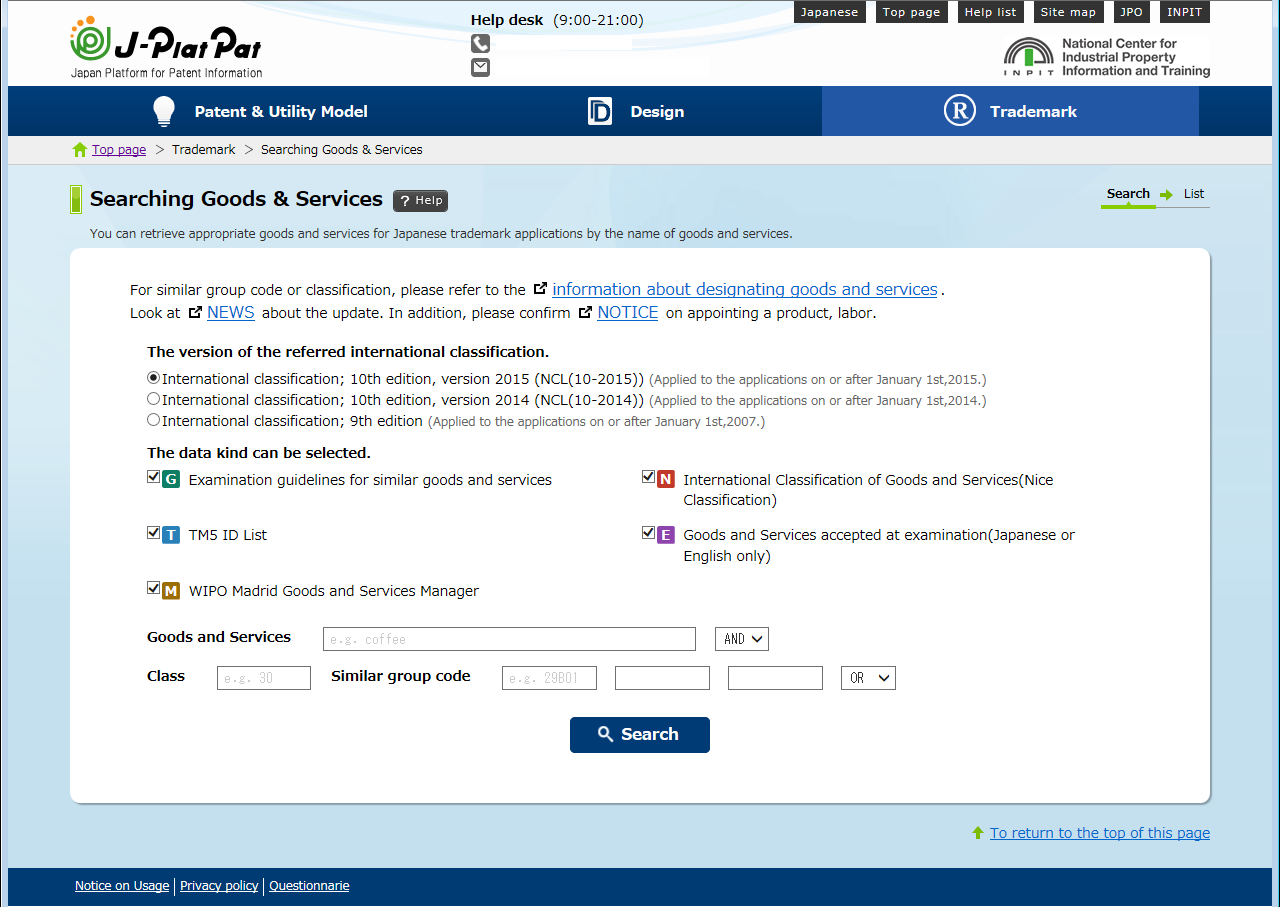Screenshot of the J-PlatPat Website Interface:

At the top of the screenshot is a white bar with a design consisting of a white swish and a blue-white-blue swish pattern. The top left corner features the J-PlatPat logo, which includes a green, swirly "J." Below the logo, the text reads "Japan Platform for Patent Information." To the right of the logo, there is text that says "Help Desk" followed by the hours of operation in parentheses (9:00 to 21:00 hours).

Further to the right, there is a colon message icon next to the text. Aligned on the top right are navigation links labeled "Japanese," "Top Page," "Help List," "Sitemap," "JPO," and "Hit," which are displayed as black buttons.

Directly below this section is a horizontal blue bar with three buttons labeled: "Patent and Utility Model," "Design," and "Trademark." Beneath the blue bar, there is a gray bar displaying breadcrumb links. The breadcrumb trail reads: "Top Page > Trademark > Searching Goods."